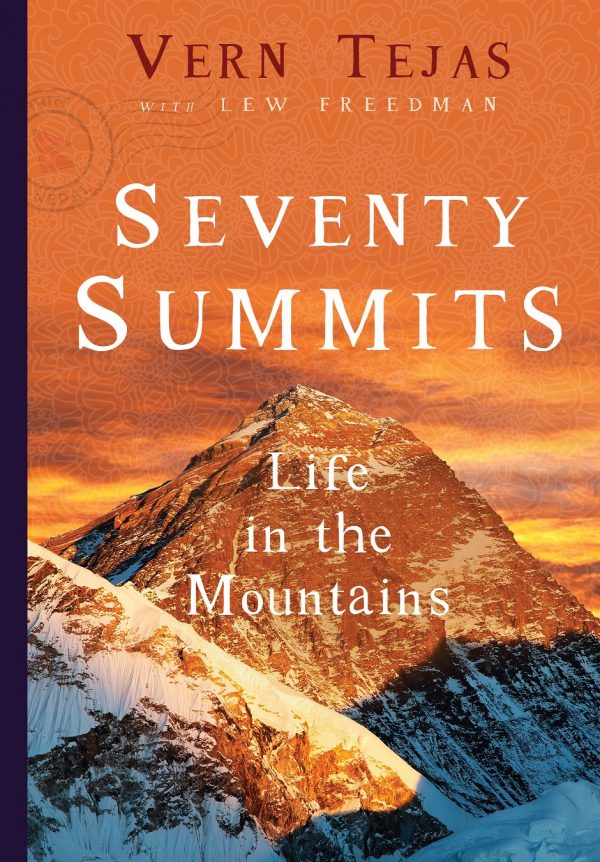The image features the cover of a book, predominantly showcasing a stunning mountain landscape. The lower half of the image captures snow-capped mountains, which gradually rise up to meet the sky, occupying the top half of the cover. As the sun sets, its orange and yellow hues blend into the mostly cloudy sky, casting a warm glow over the peaks. The book's spine is a deep purple, nearly black in color.

At the top of the cover, the author’s name, Vern Tejas, is displayed in a bold dark orange font, followed by "with Lou Friedman" in smaller white text underneath. Below this, the book title, "70 Summits," stands out in large white letters, and is supplemented by the subtitle, "Life in the Mountains," in a slightly smaller font. Adding a unique touch, a faded stamp from Nepal is visible to the left of the subtitle. The overall color palette mixes shades of orange, red, black, white, brown, off-white, and yellow, creating a visually arresting scene that encapsulates the adventurous spirit of the book.